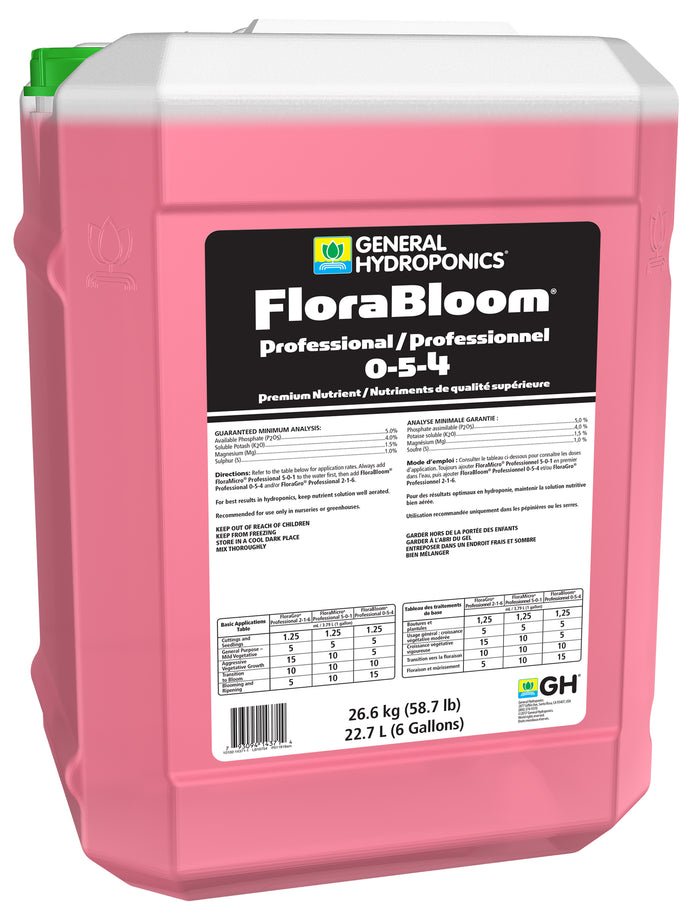This image depicts a large, pink plastic container used for gardening purposes, specifically hydroponics. The container has a distinctive green lid to the left and features an engraved image of a flower on its side. Prominently displayed on the front is a detailed black and white label. The label, crowned with a logo that includes a yellow backdrop, blue to signify water, and a red flower, reads: "General Hydroponics, Flora Bloom, Professional/Professionnel, 0-5-4, Premium Nutrients/Nutriments de Qualité Supérieure." The label contains extensive information on the product's ingredients and usage instructions, which are printed in small text alongside numerous charts and numbers. The container's dimensions are significant, holding up to 6 gallons (22.7 liters) and weighing 58.7 pounds (26.6 kilograms). A barcode is situated in the bottom left corner of the label, while another brand symbol adorns the bottom right. This detailed and aesthetically pleasing container serves as a high-quality nutrient solution for plant cultivation.